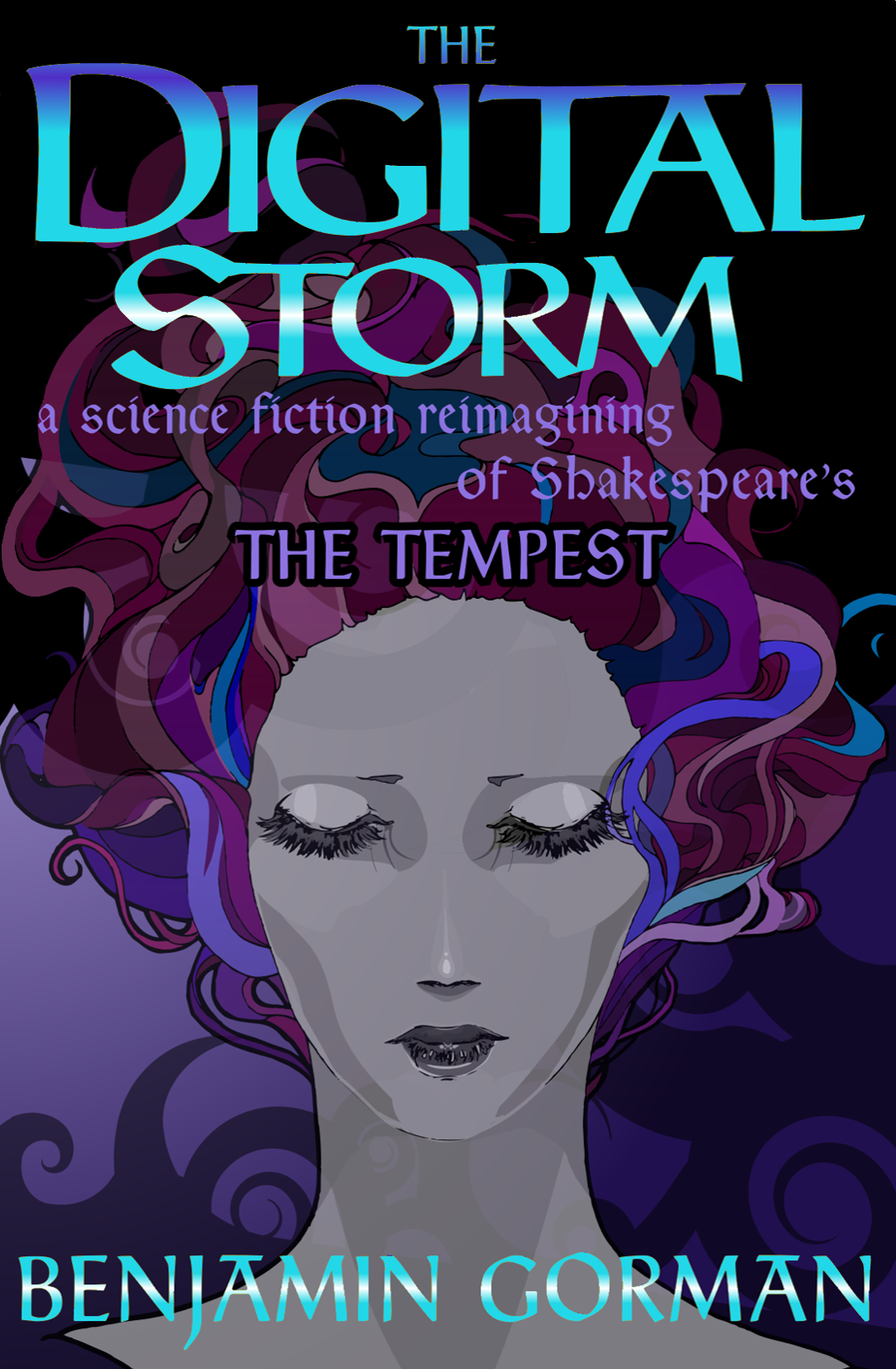The image is a vertically-oriented book cover that transitions from black at the top to deep purple at the bottom. It features a striking anime-style illustration of a young Caucasian woman with closed eyes and very long eyelashes. Her skin is depicted in shades of gray, complemented by gray lipstick and an almost nonexistent nose. The woman’s hair is a vibrant mix of reds, purples, blues, teals, and even hints of peach, cascading in wavy, flowing patterns above and around her head as though she were submerged in water.

The title of the book, "The Digital Storm," is prominently displayed at the top in turquoise letters, with 'digital' featuring a subtle purple gradient toward the top and 'storm' accented by a horizontal white light line through its center. Directly beneath the title, it reads "A Science Fiction Reimagining of Shakespeare's The Tempest" in light purple text, using a combination of fancy and blocky, all-caps fonts for emphasis. At the bottom of the cover, the author’s name, Benjamin Gorman, is also in turquoise with a white horizontal line running through the middle of the letters, matching the style of the word "storm."